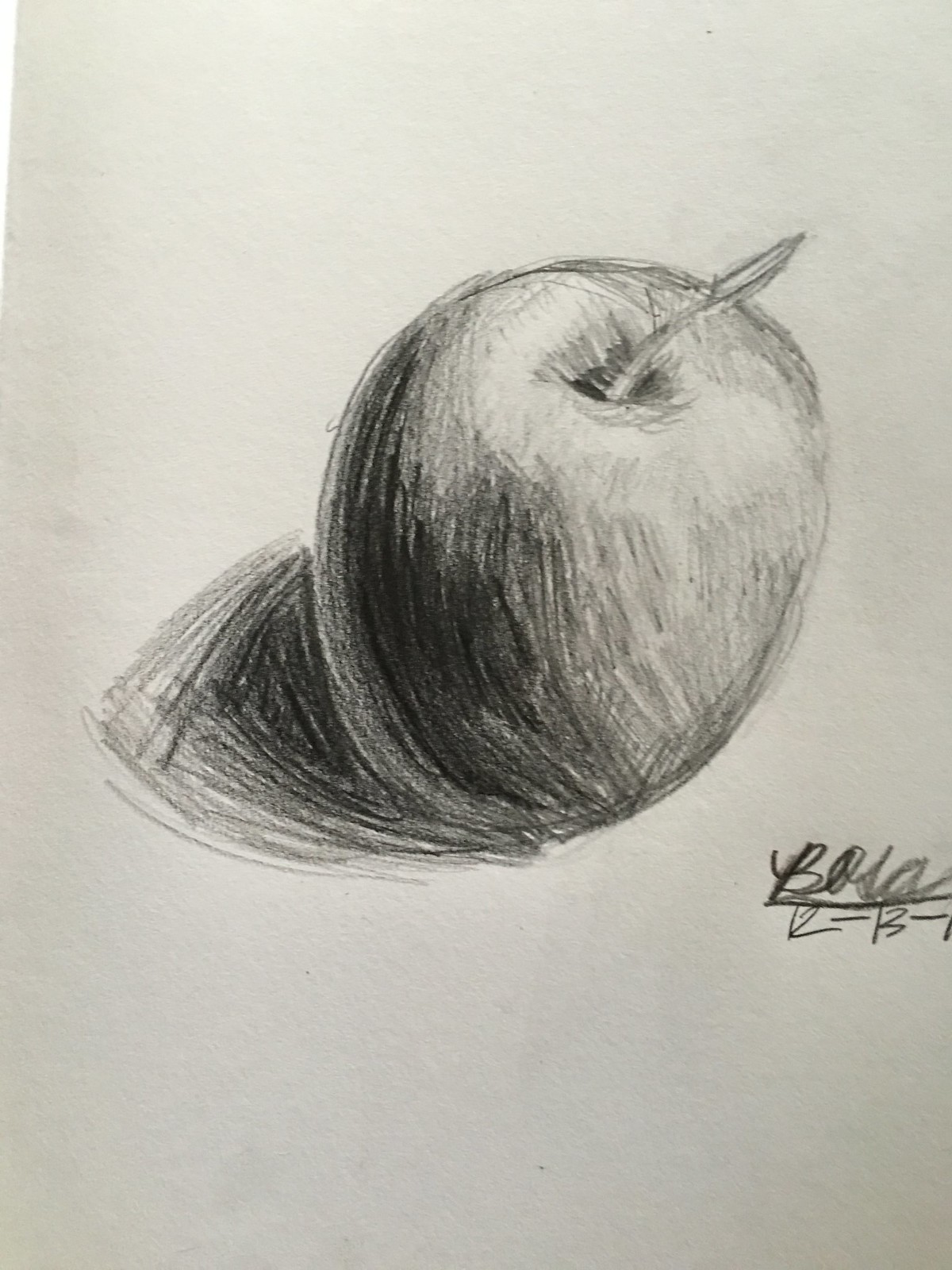Illustration Description:

The illustration prominently features an apple positioned at the bottom right corner. The apple is primarily unshaded and white, with a clearly defined stem protruding from the top. Attached to the stem is a single leaf. The left side of the apple is darkly shaded, suggesting depth and dimension, while the bottom left section also exhibits shading to simulate a cast shadow. This shading indicates that the light source is positioned on the right-hand side, casting a shadow towards the left. Above the illustration, the letters "B-O-S-A" are inscribed, and below the apple, there is an inscription that appears to read "12-13-...". The specific content of the latter part of this text is somewhat unclear.